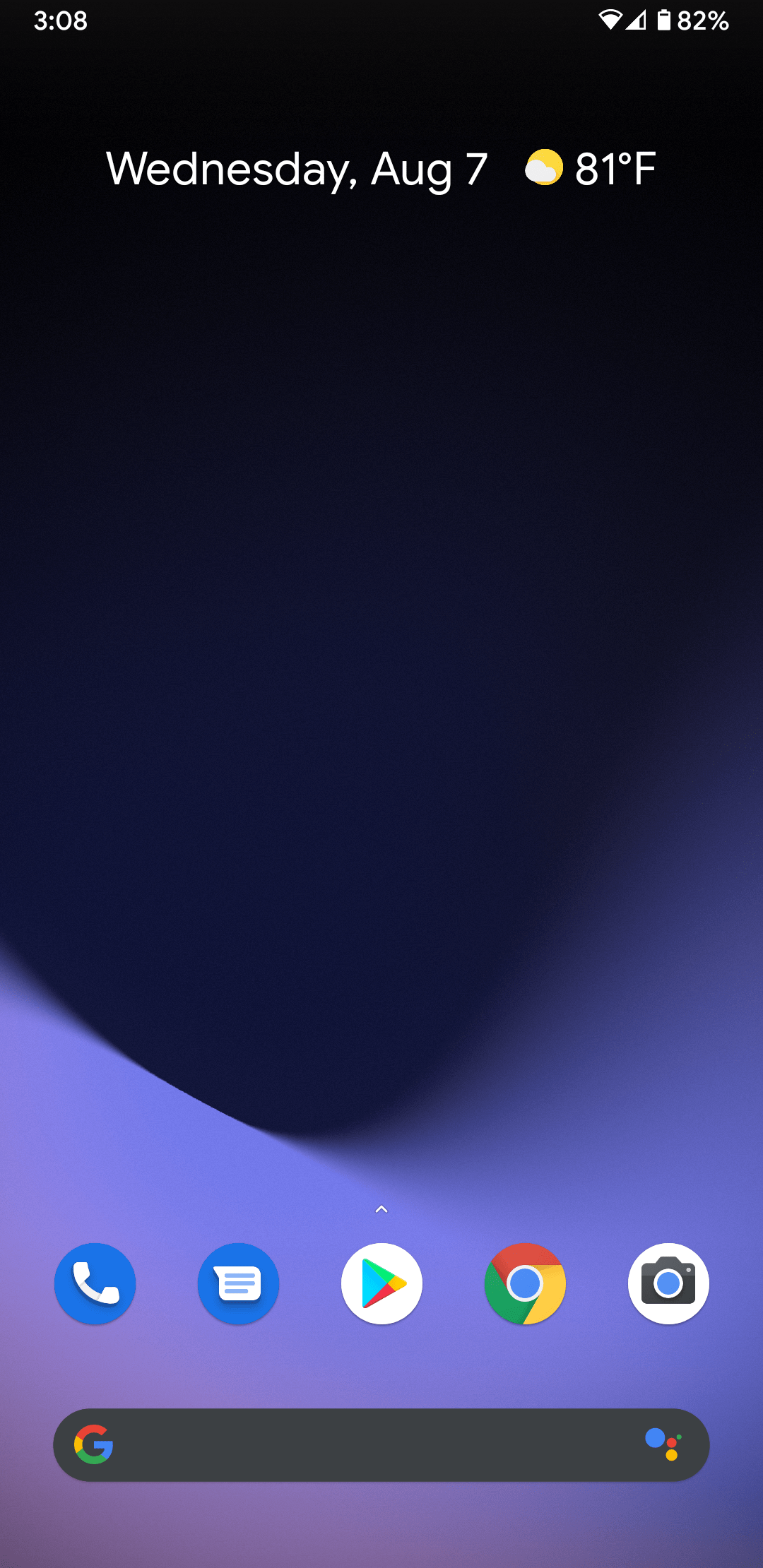The image appears to be a screenshot of an Android phone's home screen. At the top, the time is displayed as 3:08. To the right, a nearly full Wi-Fi icon and an almost filled signal bar are visible, indicating good connectivity. Next to these, a battery icon shows 82% charge.

Centered below this information, it reads "Wednesday, Aug 7," with the date accompanied by an icon of the sun partially obscured by a cloud, signifying partly cloudy weather and a temperature of 81°F.

At the bottom of the screen are five icons: a phone, a messaging app, the Play Store, Google Chrome, and a camera. Underneath these icons is a long oval-shaped search bar featuring the colorful Google "G" logo on the left and a microphone icon on the right, signifying voice search capability.

The background of the screen has a two-toned color scheme: black and violet, creating a striking visual contrast.